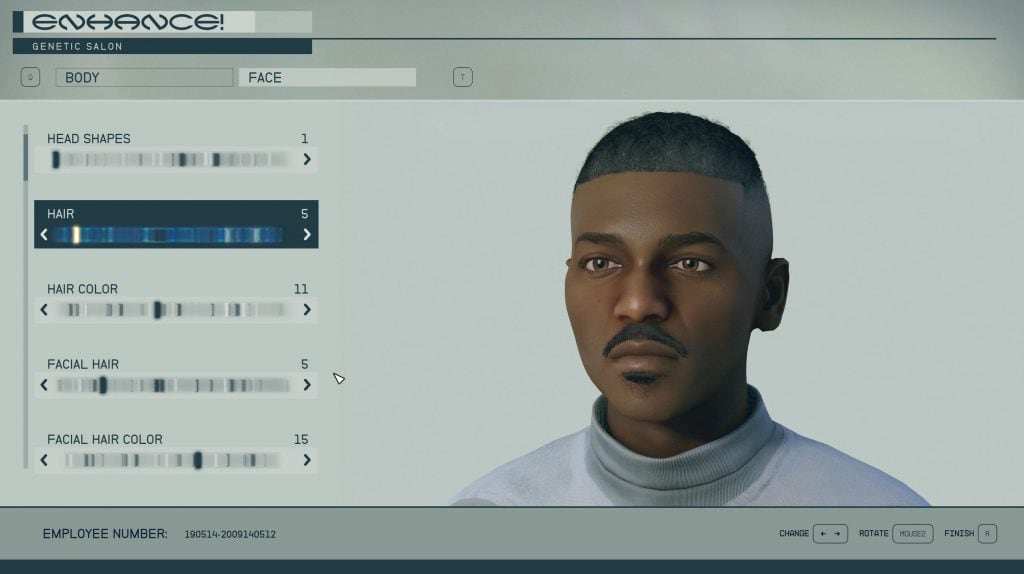The display image prominently features the word "Enhance!" in the upper left-hand corner, followed by the label "Genetic Salon." On the right side, an AI-generated image of a dark-complexioned male is showcased. He has very short hair, slightly longer on top compared to the sides, styled in a straight-edge manner. The individual sports a mustache and a small patch of facial hair just below his bottom lip. His eyes are brown, and he is dressed in a white crew neck pullover.

The interface appears to offer various customization options, as indicated by a series of controls resembling barcodes. These controls allow for adjustments in head shape, hair type, hair color, facial hair, and skin tone. At the bottom of the display, there is a section labeled "employee number," followed by specific employee identification details. Additional options available include "change," "rotate," and "finish," suggesting functionalities for modifying and finalizing the avatar's appearance.